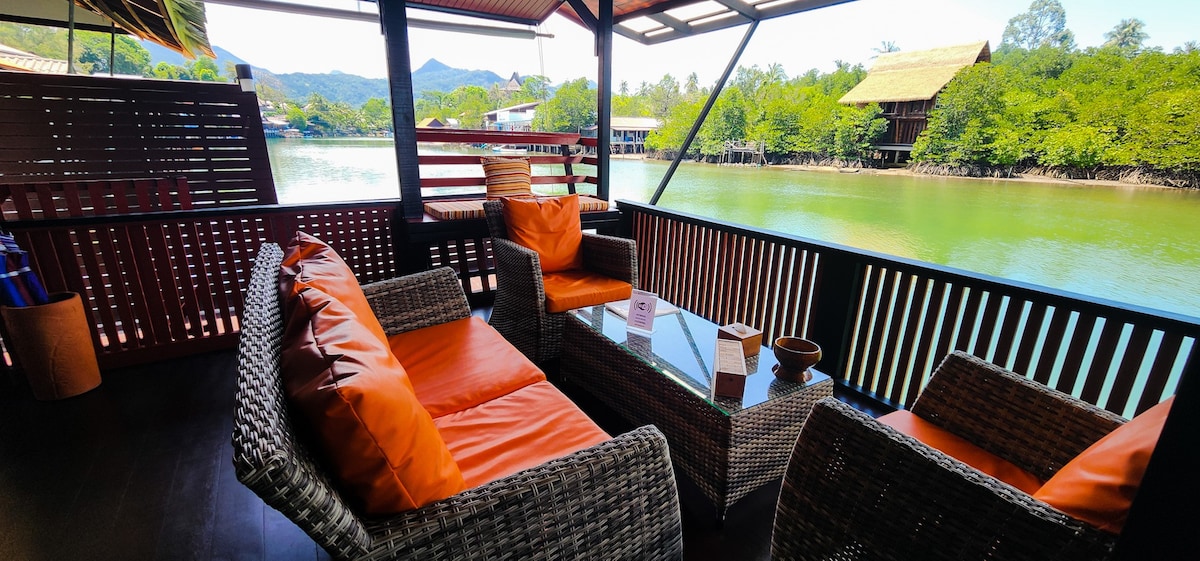In this photograph, you see an expansive outdoor patio, possibly part of a house, restaurant, or hotel, made of dark brown wood. The patio overlooks a serene body of water, which has a greenish tone, suggesting it might be a lake, pond, or river. Centered on the patio is elegant outdoor furniture constructed from intertwined wicker material in a dark brown hue, perfectly complementing the setting. The furniture includes plush, comfortable sofas adorned with dark orange cushions, and a rectangular table with a glass tabletop, creating a relaxing atmosphere. 

Adjacent to the patio, the green water body adds to the picturesque scene, which is bordered by a thick grove of trees. Among these trees, several buildings are visible, including a small shack-like structure with a light beige, sloping rooftop. In the distance, majestically towering mountains with tall peaks complete the idyllic backdrop.